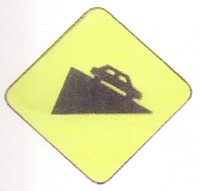The image is a small, square graphic with a predominantly bright white background that blends into areas of gray. At the center, it features a yellow, diamond-shaped road sign outlined in thin black. Inside the yellow diamond, there is a black triangle positioned on one of its sides, depicting a steep incline. Down the slope of the black triangle is a black car emblem, accentuating the warning. This straightforward design serves as a cautionary road sign to alert drivers of an upcoming hill or incline. The overall composition is minimalistic, yet effectively conveys its message with clear and simple elements.